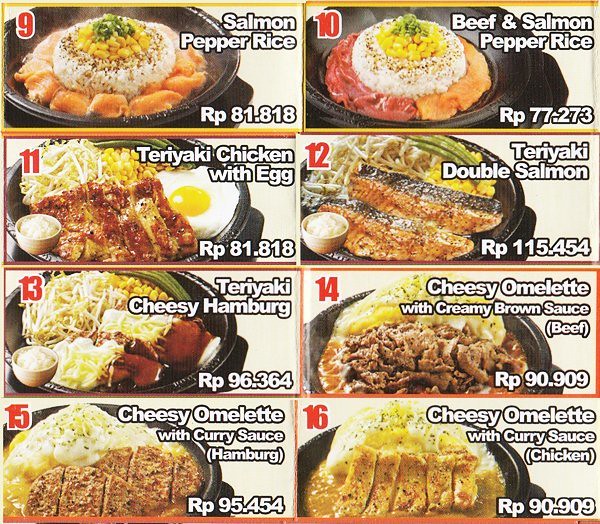The menu image displays eight dishes, arranged in two columns and four rows, with each dish depicted in vibrant, plated images. Each menu item is numbered in red, starting from 9 to 16. The left column features dishes numbered 9, 11, 13, and 15, while the right column includes numbers 10, 12, 14, and 16. 

On the top left, dish number 9 is Salmon Pepper Rice, priced at RP 81.818. The photograph shows a black circular bowl with rice in the center, surrounded by salmon slices, and topped with corn and green onions. 

In the bottom right, dish number 16 is a Cheesy Omelette with Curry Sauce (Chicken), with the price marked as RP 0.9. This dish is presented in a black circular bowl as well, featuring a yellow, cheesy omelette topped with curry sauce and accompanied by five pieces of chicken.

Overall, the menu includes diverse options like teriyaki chicken with egg, teriyaki double salmon, teriyaki cheesy hamburg, and various types of omelettes (beef, hamburger, and chicken), all vividly displayed with the meal names and their corresponding RP prices clearly marked.